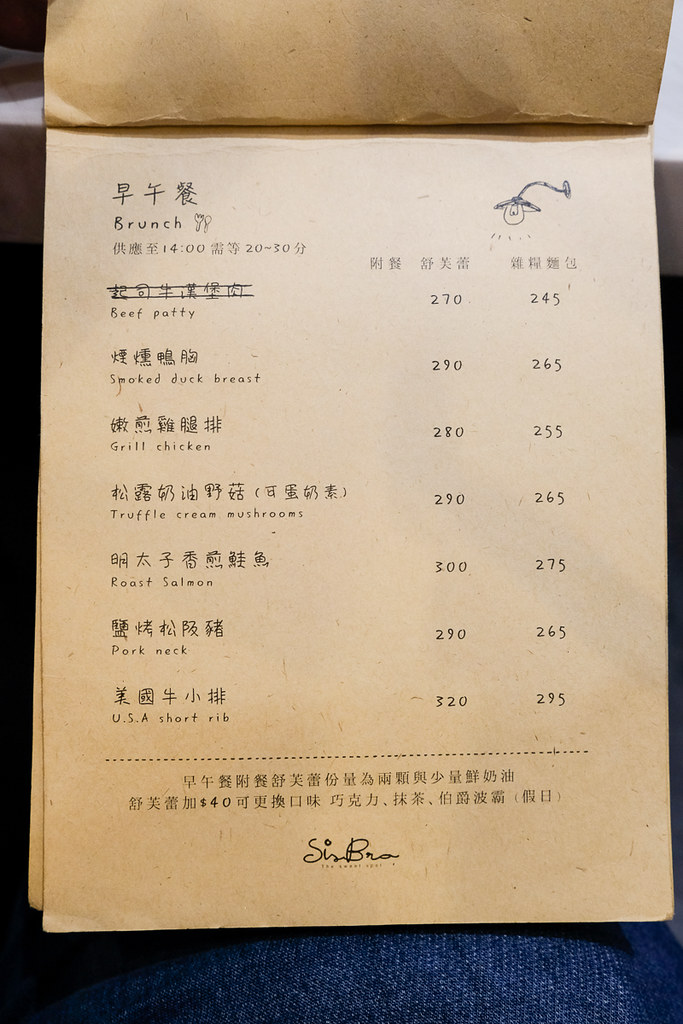This image captures a photo of a menu, presented on a standard 8.5 x 11 white sheet of paper. The menu is placed on someone's lap, with the bottom of the image revealing the dark denim of their jeans. The menu appears to be a multipage leaflet, as one page is slightly peeled upwards, hinting that it can be flipped through. The focus of the photo is on the menu itself, which is printed in black ink on white paper.

Prominently, the top of the menu features three Asian characters, followed by the word “brunch,” and a time noted as 14:00. Just below, there is a charming sketch of a light bulb emitting light from a wall. The menu lists various food options, each labeled with both Asian characters and their English translations. The English translations include items such as beef patty, smoked duck breast, grilled chicken, and roasted salmon. The prices are neatly aligned to the right of each food item descriptor.